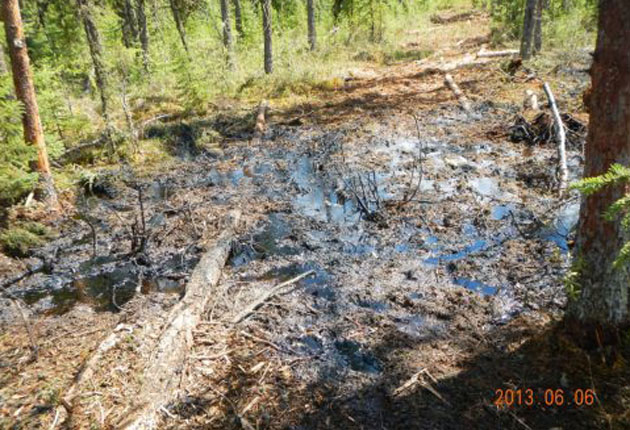The photograph, taken on June 6, 2013, captures a sunlit, isolated wooded area late in the evening. A large, swampy, muddy expanse dominates the foreground, where blue sky reflections are visible in the water, mixing with the surrounding brown muddiness. Dead sticks and twigs are scattered across this wet, boggy zone, and an old fallen tree lies half-submerged in the muck, indicating it has been there long enough for plants to grow around it. A clear dirt trail winds through the woods from the lower left towards the upper right of the image, starting beyond the swampy area and flanked by rows of green-leaved trees and brown trunks. The track appears well-trodden, suggesting it was purposefully cut through the dense foliage. Orange numbers at the bottom of the image read "2013-0606." Visitors would need to navigate through the large muddy pool to reach the other side of the trail and continue their walk through the verdant forest.